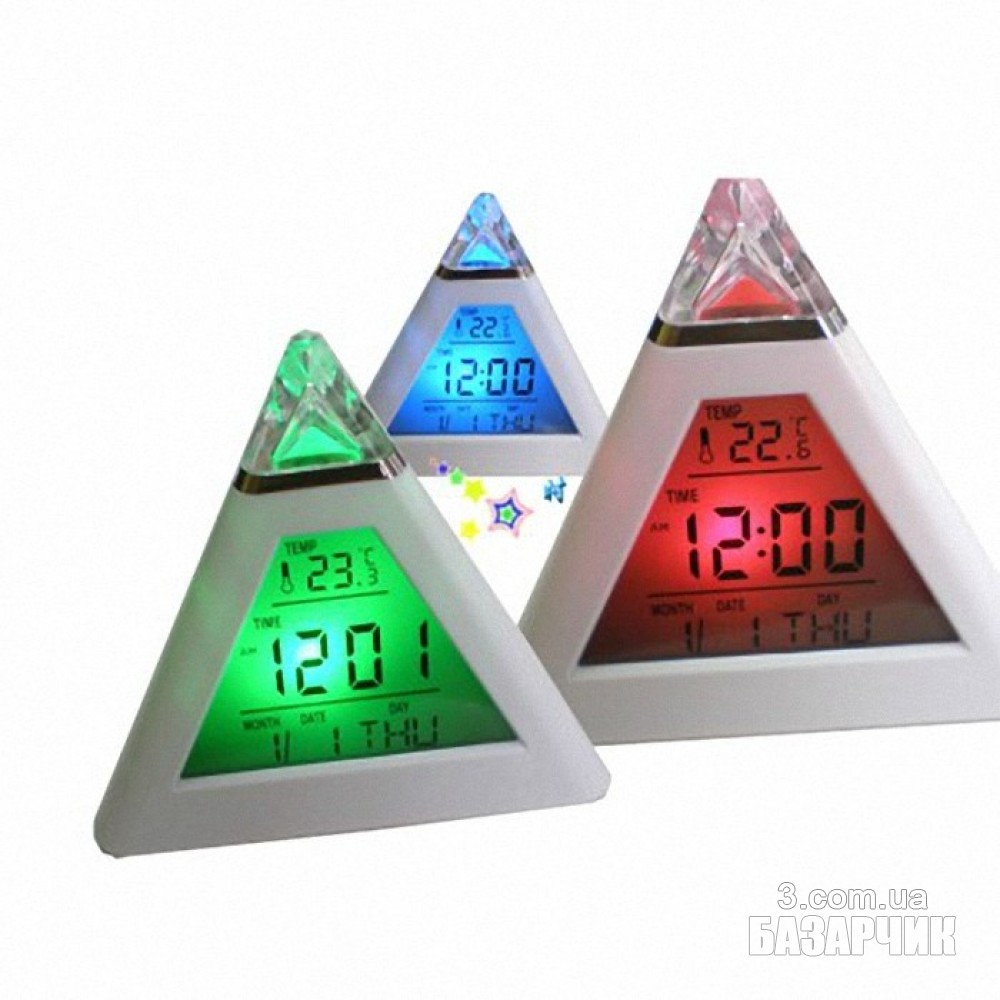Image Description: This captivating advertisement features three prominent pyramids arranged side by side against a striking background. Each pyramid has distinct characteristics and colors, contributing to the overall vividness and allure of the image.

On the far right, the red pyramid captures attention with its vibrant hue and illuminated apex. The top emits a fiery red glow, adding a dynamic and energetic feel to the scene. The text "three.com.ua" and the code "NBA3AP4NK" appear next to this pyramid, adding a unique identifier or promotional element.

The central pyramid is painted a cool blue, standing in contrast to the warmth of the red pyramid. Its face displays similar text details, including "10.3.3," "time 12," and "month and date: 1/1 Thursday." Adding to its allure, the blue pyramid features an array of sparkly stars—green, yellow, and blue—floating in front, creating a whimsical and dreamy effect.

The leftmost pyramid, predominantly white, is crowned with a crystal diamond at its peak, suggesting clarity and purity. The sign on its face is glowing, emphasizing the text "10.3.3" and other details showing time and date. The luminescent quality of the sign enhances the mystical atmosphere of this structure.

Together, these three pyramids create a visually stimulating tableau, combining elements of time, date, and vibrant colors with a touch of magical realism, making it a highly engaging advertisement.